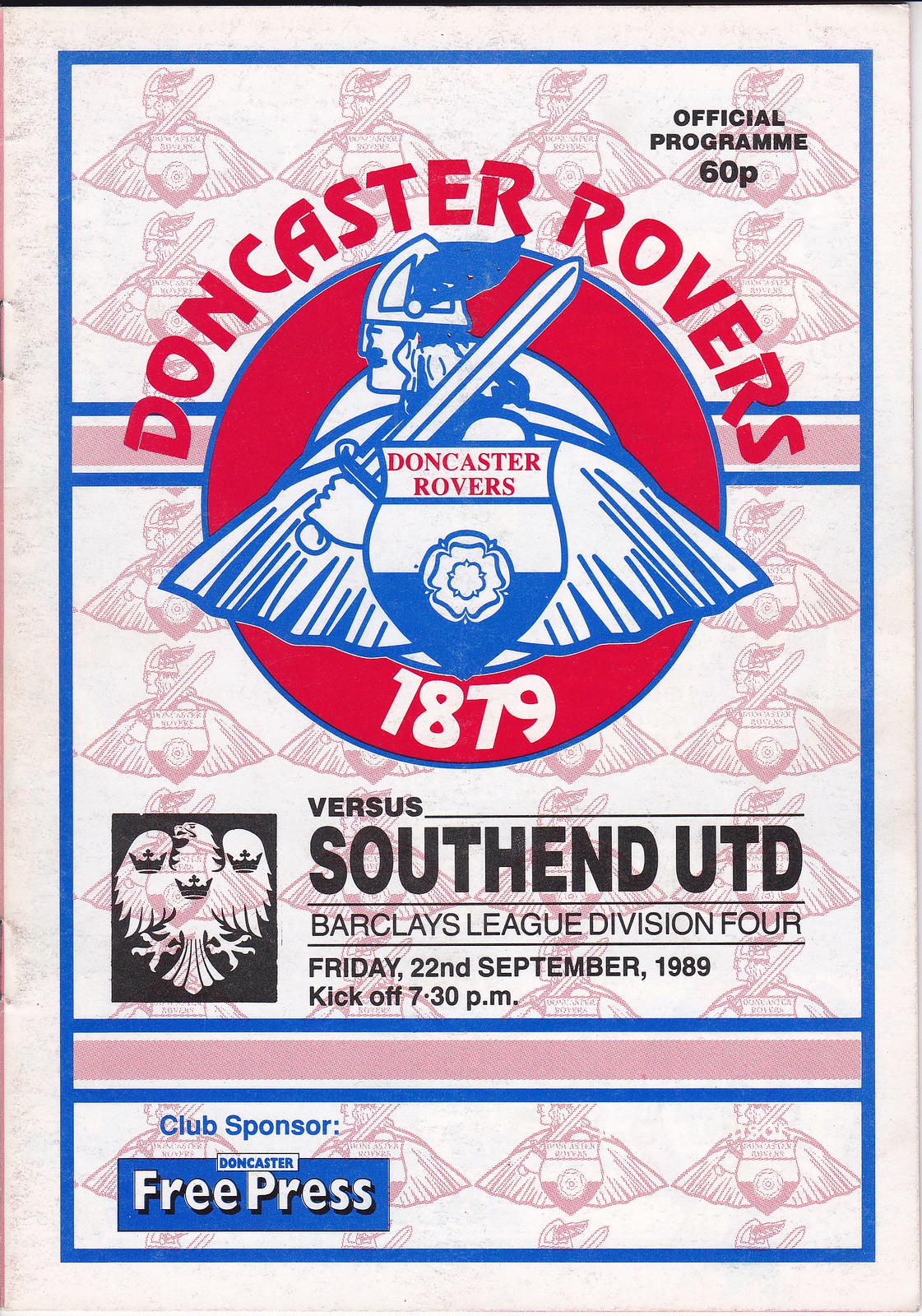This image is the front cover of an old European football program for a match between Doncaster Rovers and Southend United. In the top right corner, it states "Official Program 60p." Dominating the center of the cover, "Doncaster Rovers" is prominently displayed in large red letters. Beneath this, a red circle encloses a blue and white image of a Viking warrior with a metal helmet adorned with wings, holding a sword, and bearing a shield inscribed with "Doncaster Rovers 1879." Below this, it reads "Versus Southend UTD" and indicates it is part of the Barclays League Division 4, with the match scheduled for Friday, 22nd September 1989, at 7:30 p.m. In the bottom left corner, it notes the club sponsor, "Doncaster Free Press." The background of the cover is white, subtly decorated with a repeated grey image of the Doncaster Rovers Viking logo.